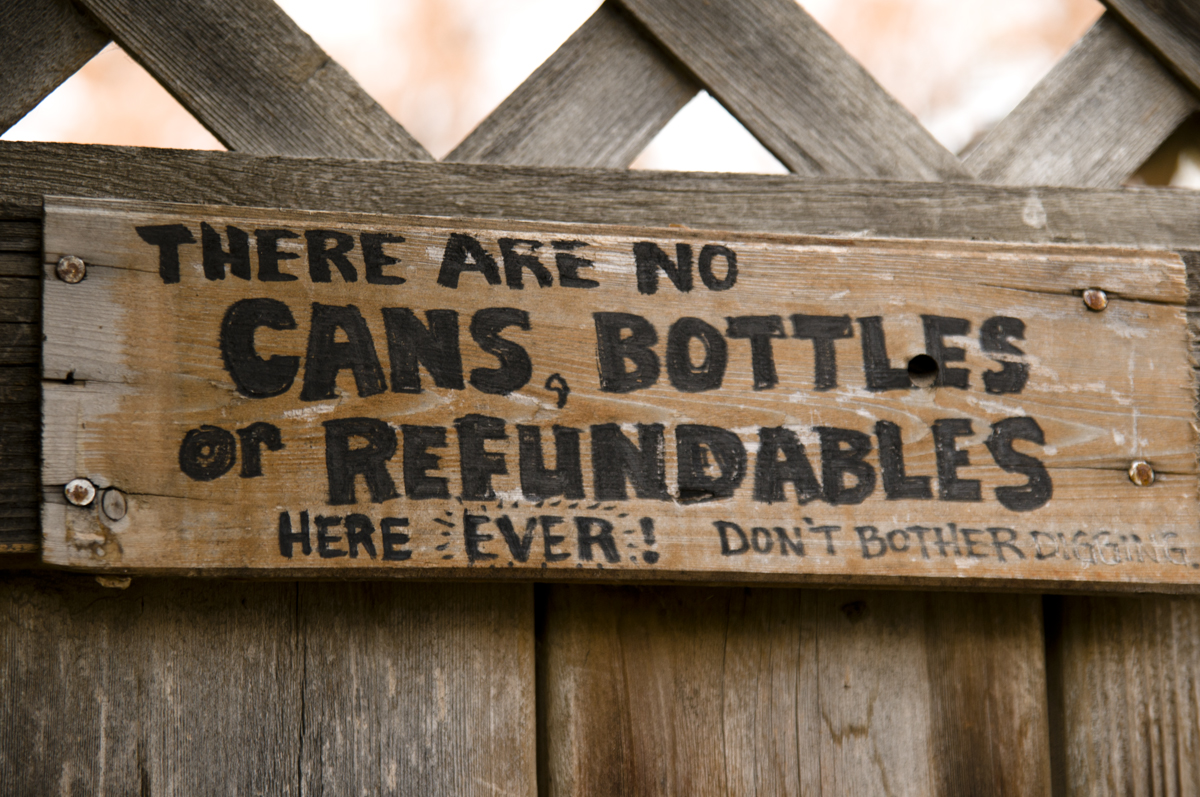This image depicts a wooden fence with a detailed hand-painted sign mounted at its center. The fence features distinctive V-shaped cutouts along the top edge. The sign, affixed with four screws that have slightly split the wood, displays a strongly worded message in all capital letters. The text reads: "THERE ARE NO CANS, BOTTLES, OR REFUNDABLES HERE EVER. DON'T BOTHER." The word "EVER" is particularly emphasized with additional marks around an exclamation point. The scene appears to be outdoors, likely photographed in the middle of the day, with the background rendered in blurred shades of brown, tan, and white, indicating sunlight filtering through.